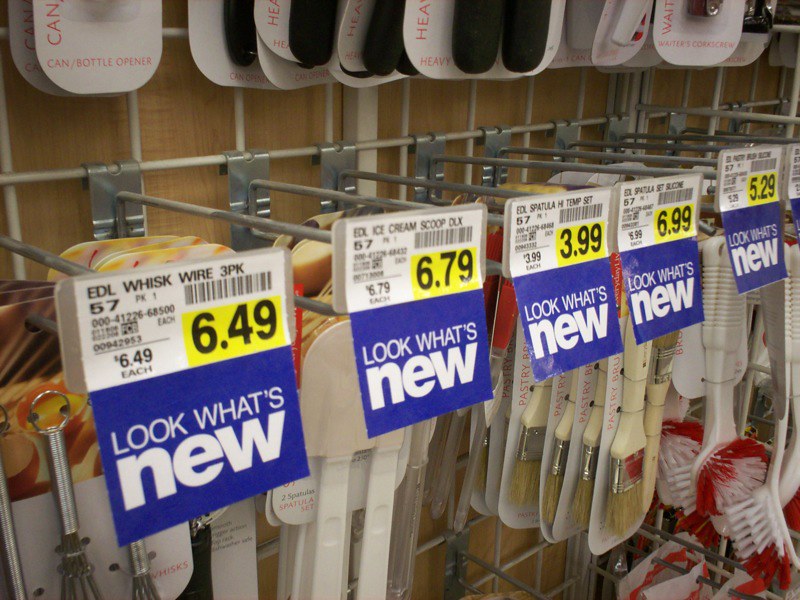This horizontal image offers a detailed close-up of an assortment of kitchen utensils neatly displayed on a metal mesh shelf. The items, mounted on long rods, include a whisk wire ($6.49 for a three-pack), an ice cream scoop priced at $6.79, a spatula temperature set available for $3.99, a basting brush, and a brush scrubber. Each item's price is prominently displayed in bold black numbers on bright yellow rectangles, enhancing visibility. In addition, large rectangular labels with white text on a blue background declare, "Look What's New," drawing attention to these fresh arrivals. The arrangement of the utensils follows a slight upward diagonal from the lower left to the upper right, adding a subtle dynamic flow to the display.